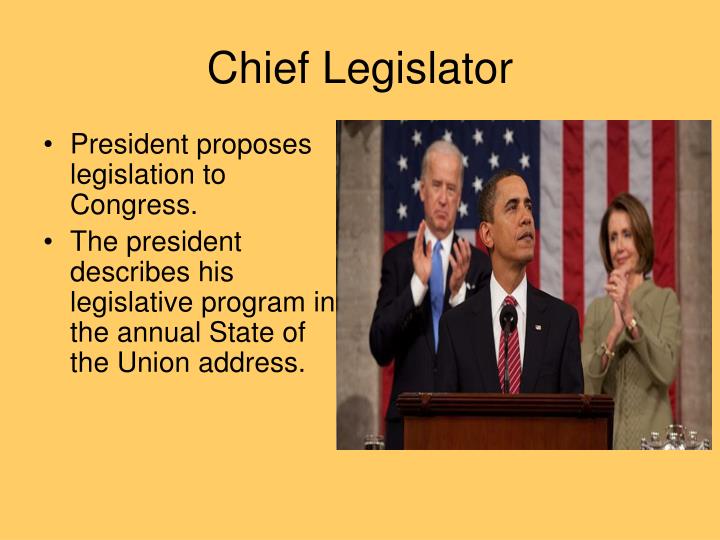The image is a horizontal, rectangular educational slide with a light yellow background, reminiscent of a presentation slide, such as one that could be created with Microsoft PowerPoint. At the top of the slide, the title "Chief Legislator" is written in a combination of black capital and lowercase letters. On the left side of the slide, two bullet points summarize key roles of the President: "President Proposes Legislation to Congress" and "The President Describes His Legislative Program in the Annual State of the Union Address."

On the right side of the slide is a photograph depicting an official event from the time when Barack Obama was President. In the image, President Obama is standing at a podium, addressing an audience, possibly in the context of a State of the Union Address given the context of the slide. Behind him, the American flag is prominently displayed. To the left behind Obama stands Joe Biden, who was the Vice President at the time, clapping. On the right side behind Obama is Nancy Pelosi, the Speaker of the House, also clapping. The photograph appears slightly grainy, and there is an indistinguishable element in the bottom right corner. Overall, the slide provides a clear and instructive representation of the President's legislative responsibilities.